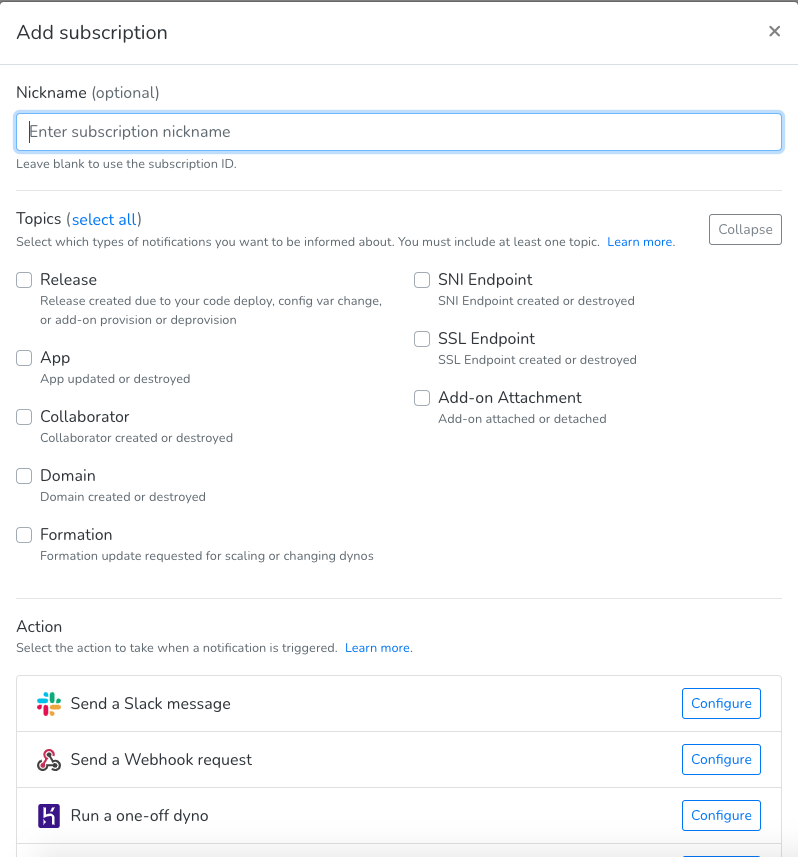**Detailed Caption:**

This image depicts a web interface for adding a subscription. The interface is titled "Add Subscription" at the top, with an 'X' icon on the upper right corner for closing the window. Directly below, there is an optional field labeled "Nickname" where users can enter a subscription nickname; if left blank, the subscription ID will be used by default.

The next section is dedicated to selecting a topic, with instructions stating "Select which type of notifications you want to be informed about. You must include at least one topic," and a "Learn More" link in blue for additional information. The main content area consists of various notification options each accompanied by a checkbox for selection. The options are detailed as follows:
- **Release:** Notifications for releases created due to code deployment.
- **Configure:** Notifications for configuration changes or additions.
- **Provision or Deprovision:** Notifications for app updates or app destruction.
- **Collaborator:** Notifications for collaborator creation or destruction.
- **Domain:** Notifications for domain creation or destruction.
- **Formation:** Notifications for formation updates requested for scaling or changing dynos.
- **SNI Endpoint:** Notifications for SNI endpoint creation or destruction.
- **SSL Endpoint:** Notifications for SSL endpoint creation or destruction.
- **Add-on Attachment:** Notifications for add-on attachments or detachments.

On the right side, there is a "Collapse" button that allows users to hide detailed options. Below the topic selection, there is an "Action" section where users can select the action to be taken when a notification is triggered, along with another "Learn More" link for further guidance. The interface predominantly uses a dark gray font with blue highlights for interactive elements.